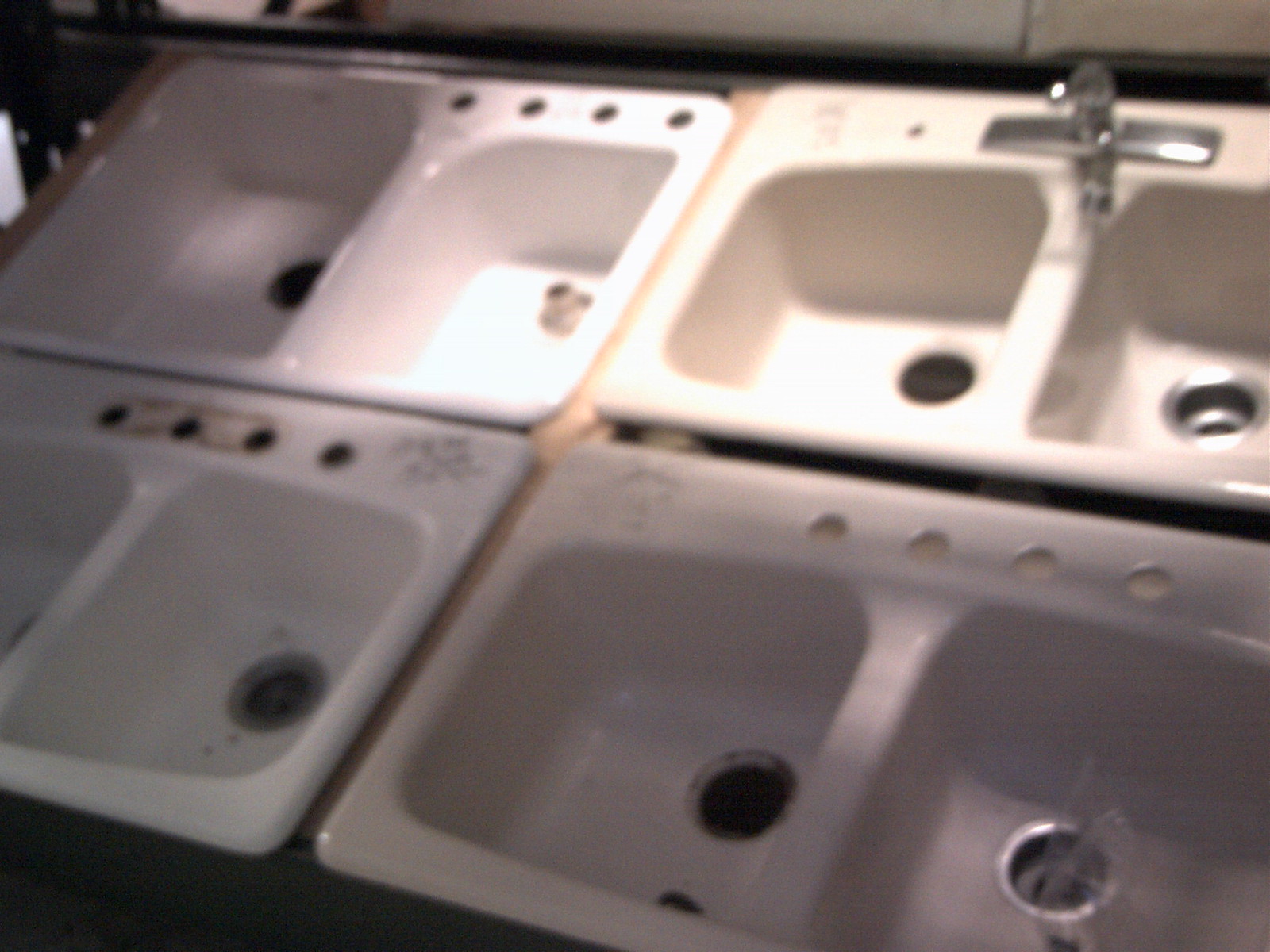A blurry photograph captures four old, double-basin sinks arranged in a grid with two on the top and two on the bottom. The angle of the shot makes the left-side sinks appear slightly smaller. Each sink is divided into left and right sections, with a drain near the middle divider. The top left sink has metallic-looking objects protruding from the right drain. The top right sink features a single-handle, silver faucet with a rotating nozzle, while the other sinks are missing their hardware. The bottom left sink shows significant rust and staining around the faucet holes. The sinks are mostly white, although the top right and bottom left ones appear off-white or beige. Plastic seems to be protruding from the drain of the bottom right sink. Overall, the primary colors noticeable in the image are white and silver.